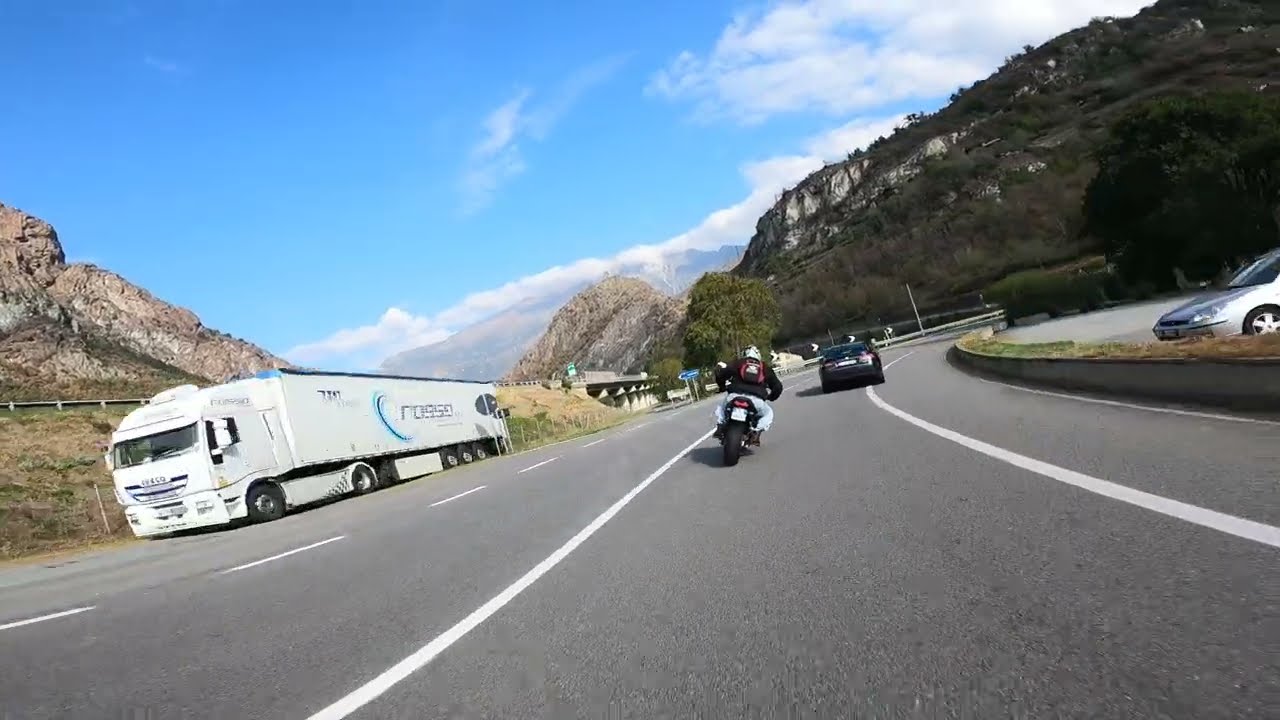The image captures the perspective of a motorcycle rider traveling on a multi-lane highway, framed by a scenic landscape. The asphalt road, marked with solid white lines on both sides and a dashed white line in the center, stretches forward before curving slightly to the left and dipping under a bridge supported by columns. 

Ahead on the right lane, another motorcycle is leaning slightly to the right, ridden by an individual in a black jacket, light blue jeans, and a two-color helmet, carrying a black and red backpack. This motorcycle trails a black car, while a white semi-truck with "ROSSO" and a blue half-circle emblem on the side occupies the left lane.

To the far right, a silver car is parked near a barrier that separates the road from a parking lot. The distant landscape features a rocky mountain with sparse vegetation and a prominent, leafy green tree in the middle ground. The upper left corner of the image showcases a partly cloudy blue sky, capturing the setting of an outdoor, mid-day journey on a winding highway.